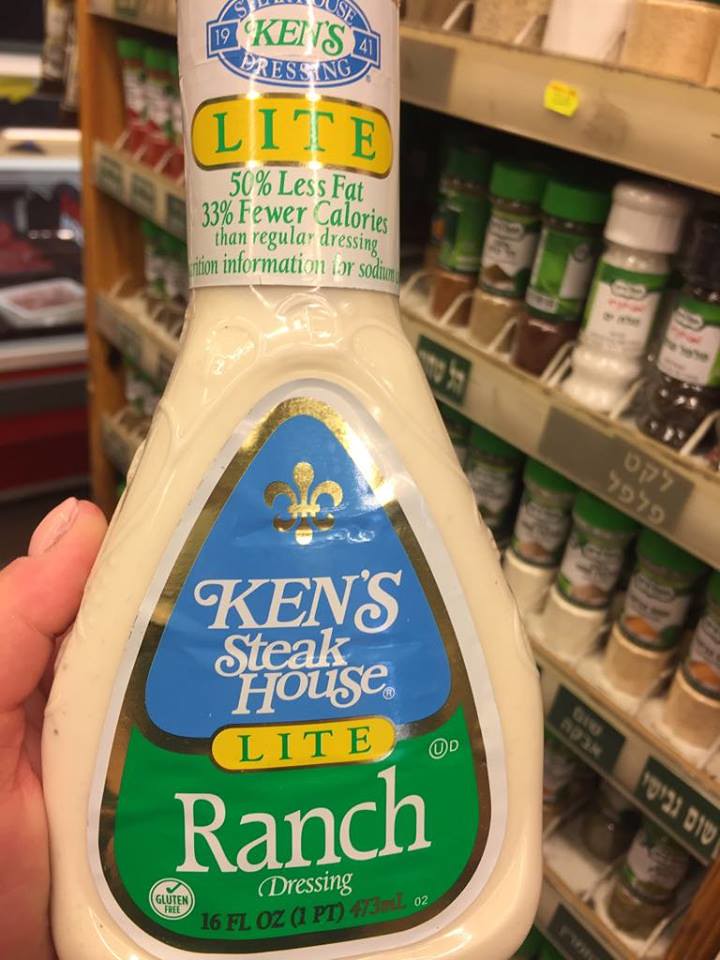This color photograph, taken indoors, captures a close-up of a person's left thumb holding a bottle of Ken's Steakhouse Light Ranch Dressing. The bottle is primarily white, wide at the bottom, and tapers towards the middle with a tall neck. The neck features a white label with green text that reads "Ken's Light," highlighting "50% less fat" and "35% fewer calories than regular dressing," followed by some information about sodium content. The main label on the front of the bottle has gold edging and displays "Ken's Steakhouse Light Ranch Dressing" in white text against a blue, green, and yellow background, along with a crown emblem at the top. The bottle's capacity is noted as "13 fluid ounces (2 pints, 673 millilitres)" in black text. In the background, multiple shelves filled with jars of various foodstuffs, predominantly in white, green, and brown, are visible, with beige-colored shelves and a metal tray containing beige food items in the upper left corner.